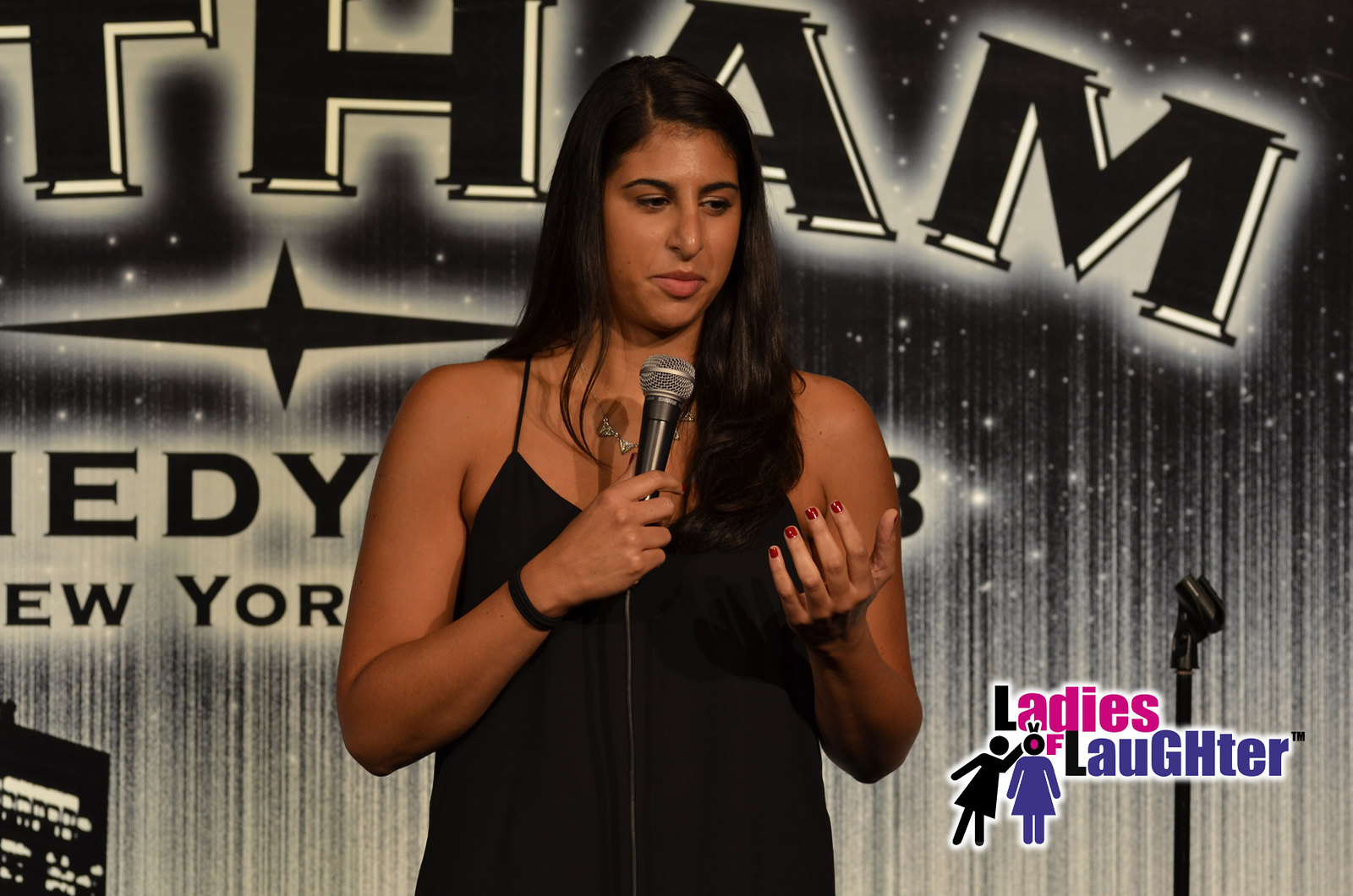The image is a poster or advertisement card showcasing a comedian at a stand-up show, most likely set in New York, based on the partial text visible in the background. The photo captures an indoor setting with a black and white curtain adorned with sparkles and lights. The main subject is a young woman, possibly white or Hispanic, with somewhat dark skin and long black hair falling past her shoulders. She is wearing a black spaghetti strap tank dress and is holding a silver microphone, which has been detached from its stand that remains visible to her left. Her red-painted nails and a black bracelet on her right wrist stand out as she addresses the audience, looking slightly down. The background features incomplete letters "T-H-A-M" and "E-D-Y," suggesting it might say "Gotham Comedy, New York." In the bottom right-hand corner, there is a graphic of two women and the text "Ladies of Laughter," reinforcing the comedic theme of the event.